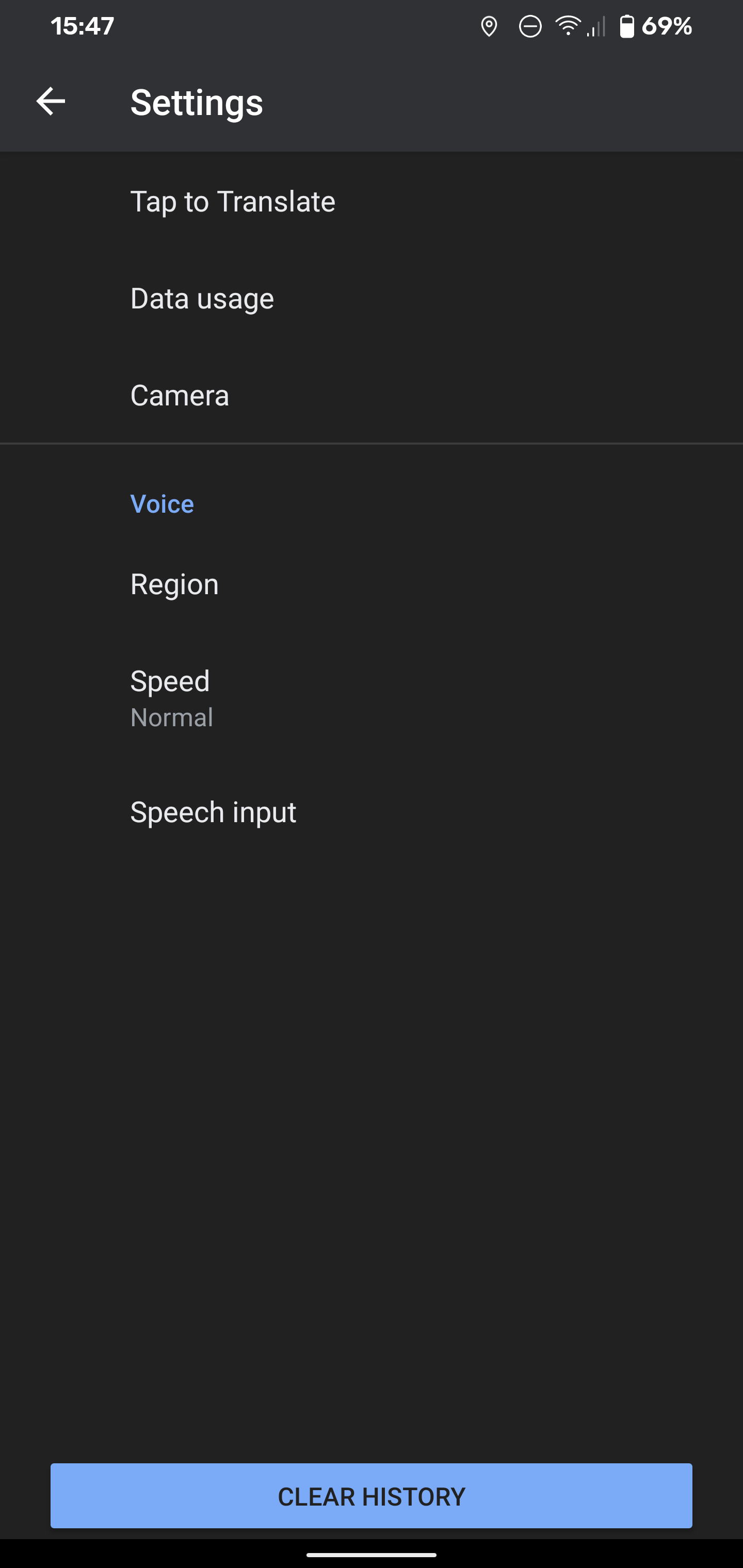The image shows a screenshot of a mobile device's interface with various system information and settings displayed. In the top left corner, it indicates the time as 15:47, followed by icons displaying a PIN symbol, a circle with a minus sign, a Wi-Fi signal with 2 out of 4 bars, and a battery icon showing 69% charge. Adjacent to these icons, there is a back arrow symbol and the settings icon.

Below this header, there are several menu options: "Tap to Translate," "Data Usage," and "Camera." These options are listed in a line, suggesting quick access features. Additionally, there is a section highlighted in blue containing options for "Voice," "Vision," "Speed," "Normal," and "Speech Input." The background of this section is darkened, making the blue options stand out prominently. 

At the bottom of the screen, there's a blue rectangle button labeled "Clear History," alongside a red button represented as a dark rectangle with a dash, which might suggest a delete or clear function. Overall, the screen displays a mix of system status indicators and functionality shortcuts, with certain elements emphasized for user convenience.